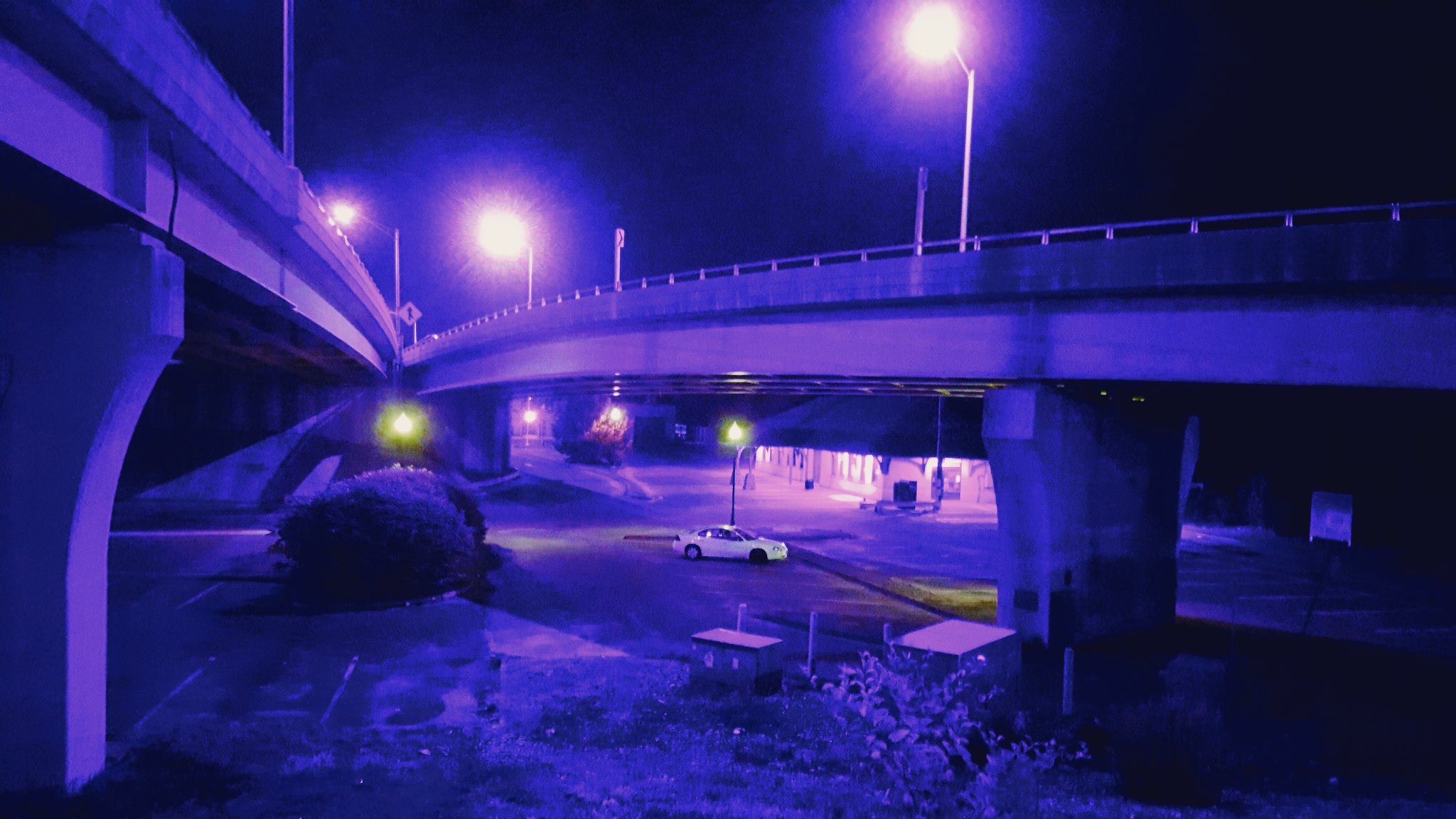This color photograph, taken at night in landscape orientation, captures a striking scene of two flyover bridges viewed from below, converging toward the horizon from the right and left sides of the image. The top half of the photo is dominated by a dark black sky accentuated with lavender rays of light, likely enhanced by a heavy filter that casts a purple glowing hue across the entire scene. 

Underneath the converging bridges, amidst a parking lot, a solitary white sedan is prominently featured. This car is parked to the right and conspicuously missing a hub cap on its front tire, which reveals a black tire. The back tire, however, retains its hub cap. Surrounding the car, the scene is illuminated by seven street lamps casting a surreal purple light.

In the center-left of the photograph, a large bush grows on the pavement, with additional shrubbery and two small white pillars visible in the foreground. Moreover, several traffic lights are discernible behind the car, and the roads stretch into the distance. The overall effect is one of photographic representational realism, making the surreal night setting both vivid and tangible.